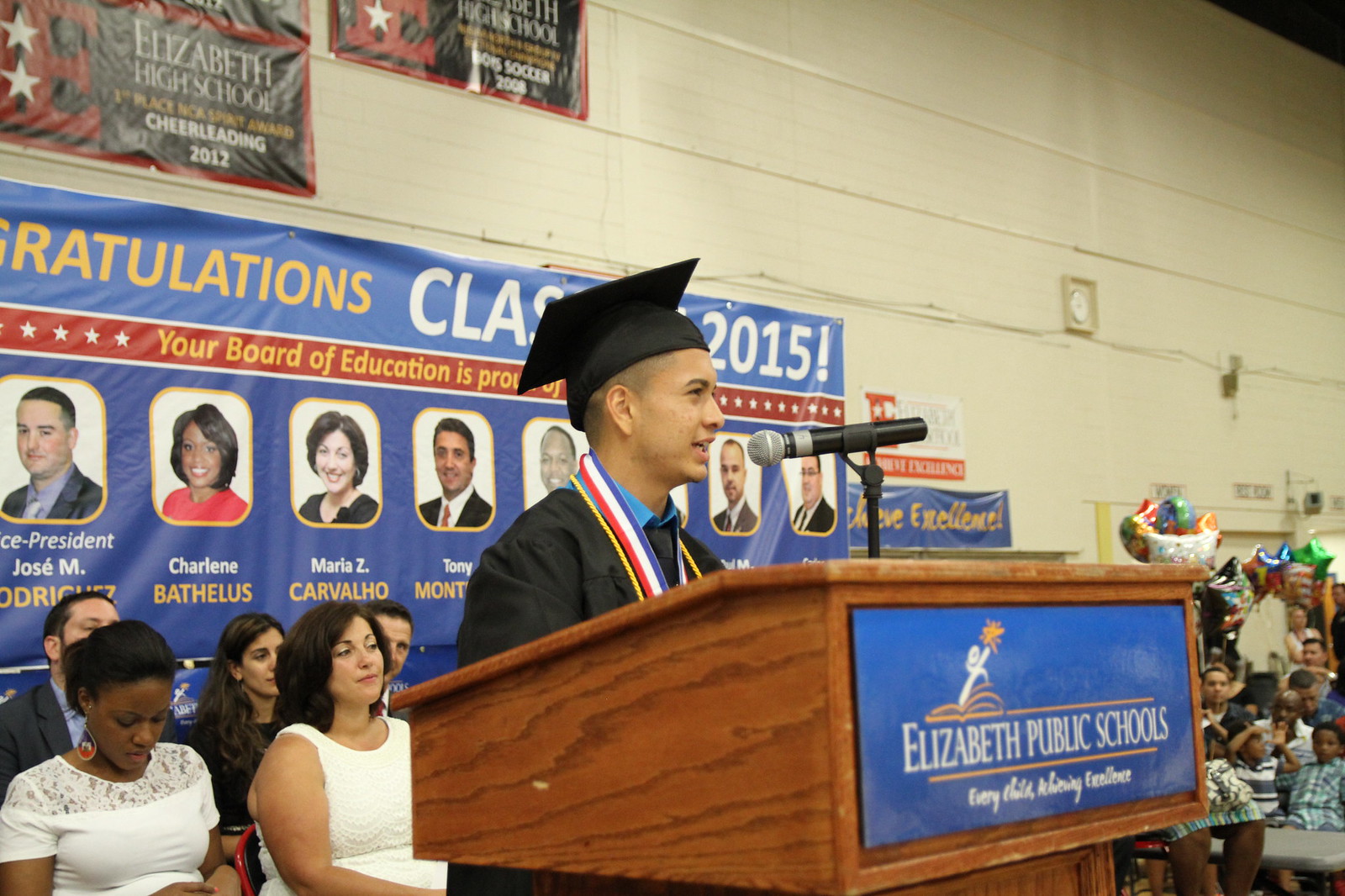The image captures a vibrant graduation ceremony held in an auditorium or gymnasium, where a young man adorned in a black graduation cap and gown, accented with honor cords and ribbons, stands at a wooden lectern. The lectern boasts a blue sign with the words "Elizabeth Public Schools: Every Child Achieving Excellence" inscribed in white letters. The graduate is speaking into a microphone, delivering what seems to be an important part of the ceremony.

Dominating the background is a large banner that reads, "Congratulations Class of 2015," partially obscured by the speaker's head. This banner also includes photos of the Board of Education and a message that reads "Your Board of Education is proud of," though the rest of the message is not visible. To the left behind the speaker, several individuals—likely other speakers or diploma presenters—are seated, whereas the lower right corner of the image reveals numerous audience members holding helium balloons and shiny celebratory items, adding to the festive atmosphere. The setting features a beige brick wall, providing a backdrop to this momentous occasion.